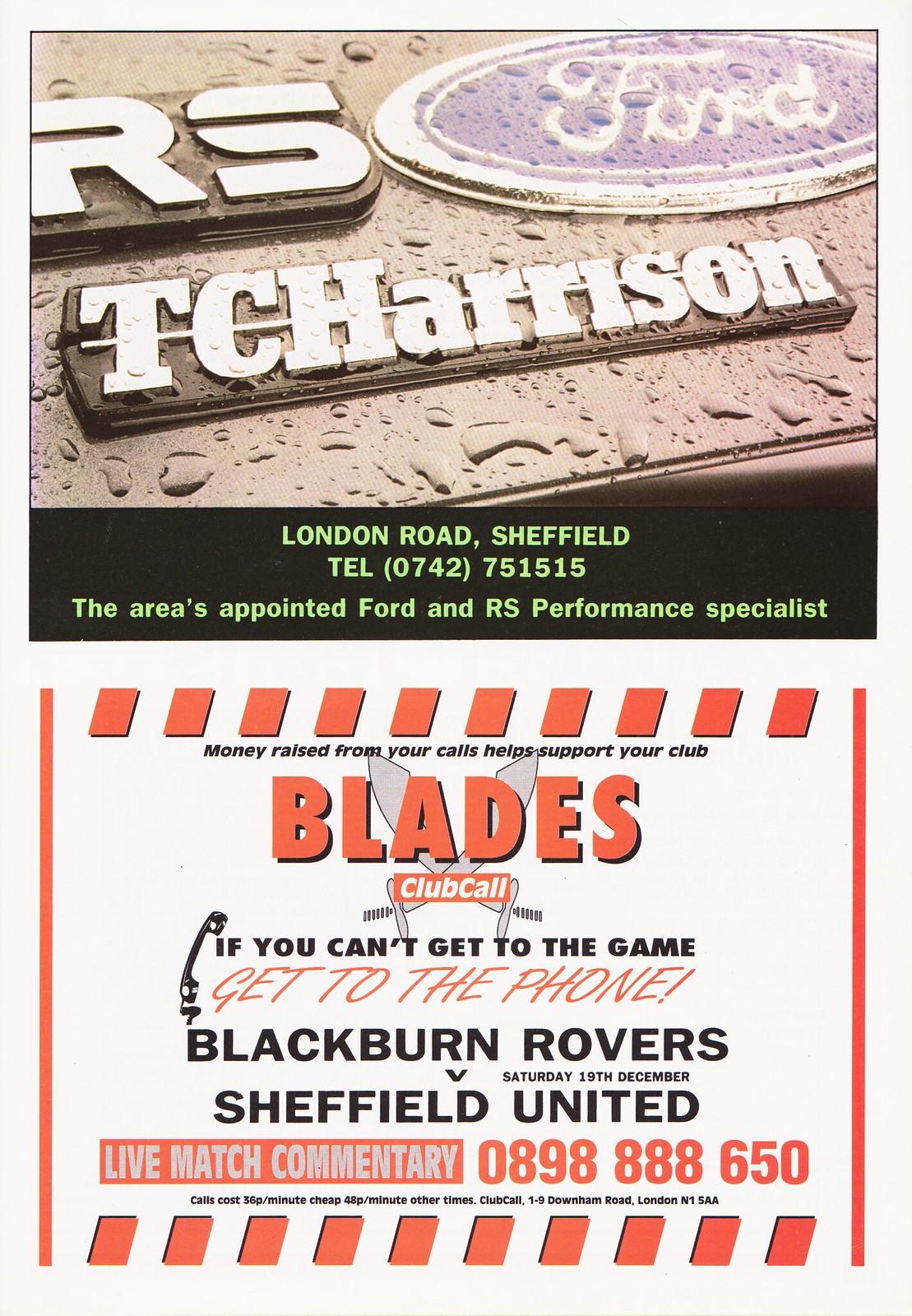This vertically aligned rectangular ad, seemingly for a local Ford dealer on London Road in Sheffield, UK, features two prominent sections. At the top, a square section displays the Ford logo within an oval shape with a silver border, alongside the initials "RS." Below it reads "T.C. Harrison" followed by "London Road, Sheffield" and a telephone number: 0742-751515—all in light green text against a black background. This section highlights that the area is an appointed Ford and RS performance specialist.

The lower section of the ad transitions to a sports theme, prominently featuring "BLADES" in large red all-caps letters. It encourages fans with the slogan, "If you can't get to the game, get to the phone." This part promotes a Club Call service for live match commentary of the Blackburn Rovers versus Sheffield United soccer match on Saturday, 19th December. The black text sits on a red rectangular background, providing the contact number 0898-888-8650 for donations, emphasizing that money raised from these calls supports the local soccer club. The overall color scheme and detailed descriptions in both sections indicate a blend of automotive sponsorship and fervent community sports support.